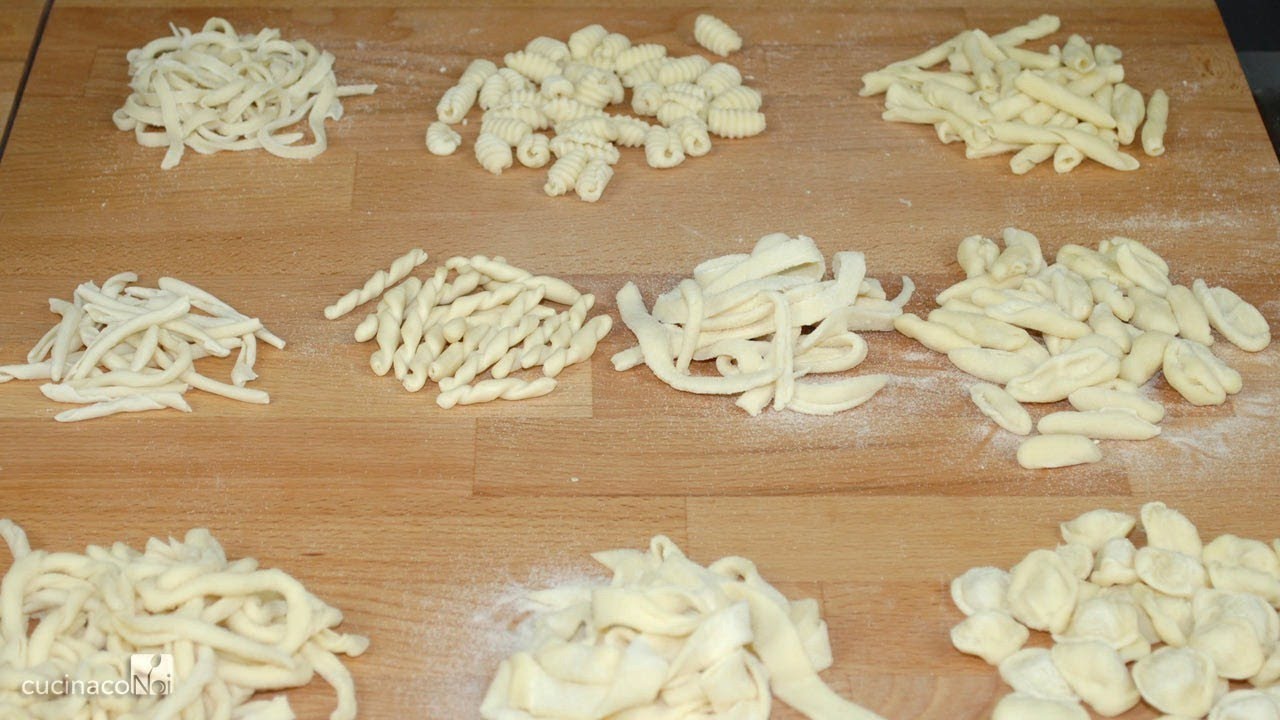This detailed color photograph, taken in landscape orientation, showcases a light brown wood cutting board or tabletop covered with various piles of homemade pasta. The image captures a view looking slightly downward, featuring a total of ten distinct piles of raw pasta: three at the top, four in the middle, and three at the bottom. The uppermost row includes wide fettuccine noodles, corkscrew-shaped pasta, and penne. The middle row contains four different types of pasta, while the bottom row mirrors the top with three more piles. Each variety of pasta, including fusilli, gnocchi, rigatoni, capeletti, and ravioli, displays a light creamy beige color, indicative of a dough with minimal yolk content. A light dusting of white flour is scattered around the piles, emphasizing the homemade nature of the pasta. The photograph also features an inscription in the bottom left corner with the text "Kuchinako" and a white square containing the letters "NOI". This image exemplifies photographic representationalism, focusing on realism and food photography to highlight the delicate textures and shapes of the pasta.